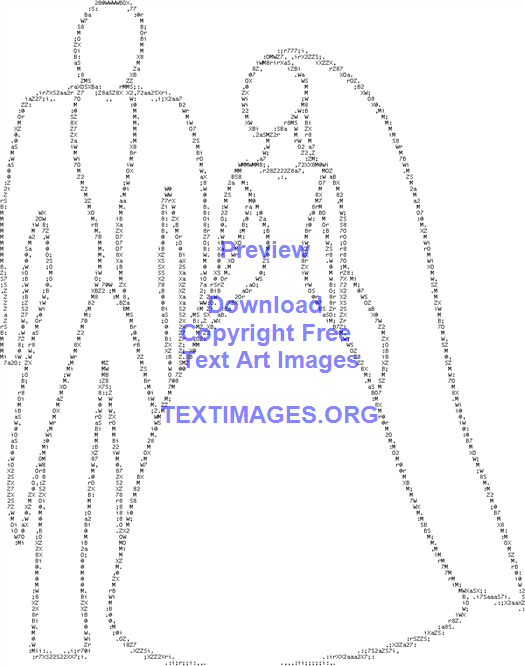This image is a detailed ASCII art sketch, featuring a groom and a bride. The figures are meticulously constructed using very tiny, almost imperceptible characters, including letters, numbers, and symbols, that form a pattern resembling a groom in a suit on the left and a bride in a voluminous dress with a long veil on the right. The outlines are simple and general, devoid of any facial features or textures in their clothing, with the bride's veil flowing from her headpiece to the floor. The background is plain and white, providing a stark contrast that highlights the minimalistic yet intricate text-based artwork. At the top of the image, blue text reads "preview, download copyright free text art images, textimages.org."